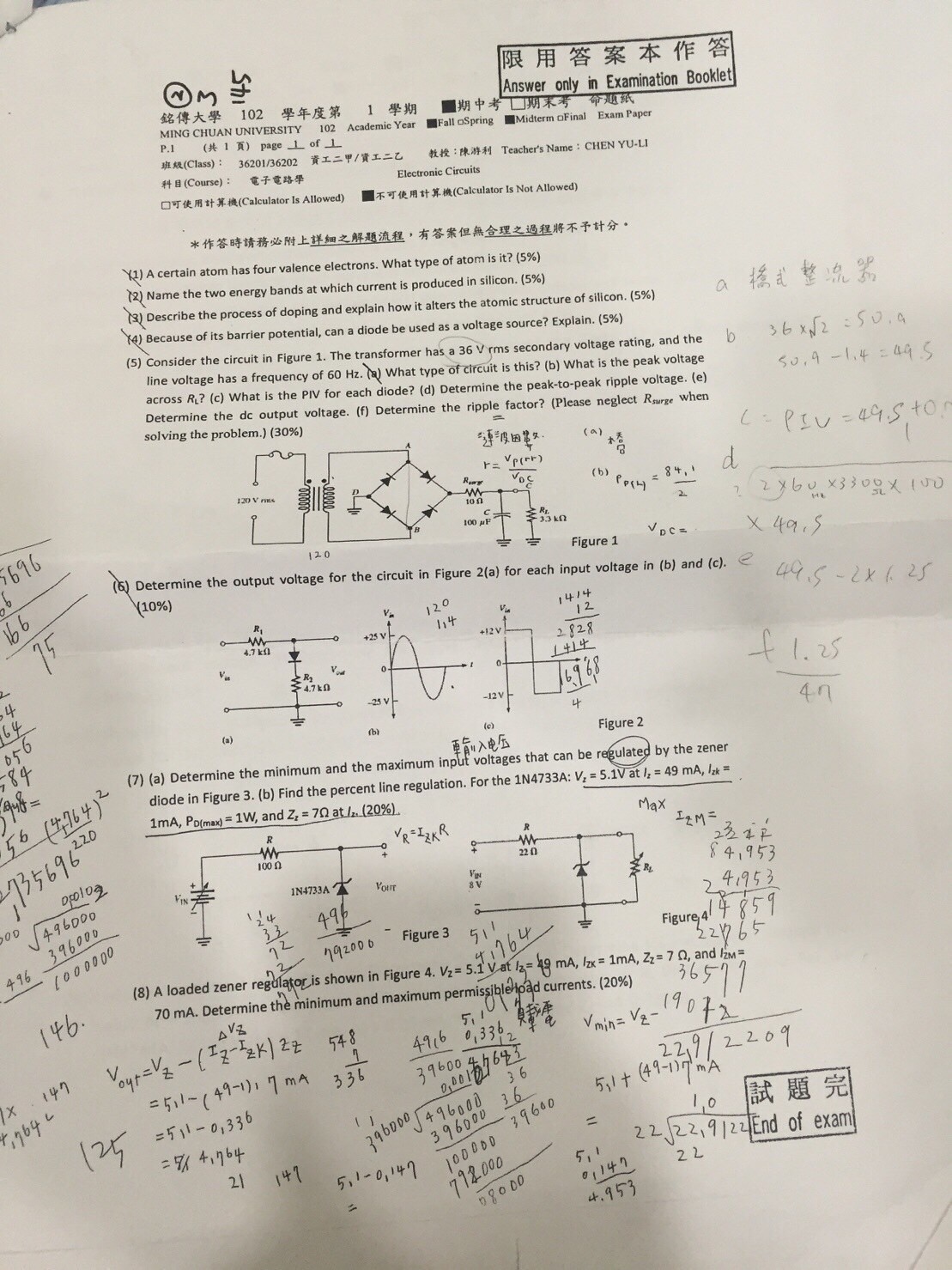This is a vertical, rectangular, black and white test page from a college, possibly Ming Tuan University, for the academic year 102, fall semester midterm exam. The page has a grayish-white background with centered text at the top indicating the university name and exam information, including phrases like "Answer only in examination booklet" and various Asian characters. The page features a series of eight questions that cover topics such as the identification of atoms with specific valence electrons, energy bands in silicon, doping processes in atomic structures, uses of diodes based on barrier potential, and circuit analysis with accompanying figures.

The layout includes multiple black text sections interspersed with diagrams and computations. Handwritten mathematical equations and notes in both pencil and pen are present along the edges of the paper, particularly on the right side and bottom, indicating someone actively worked on the problems on this sheet. At the bottom right corner, there's a black rectangle stamp with Asian characters and the phrase "End of Exam," reinforcing the conclusion of the test. The overall design is meticulous, suggesting an official academic document used for student evaluations.